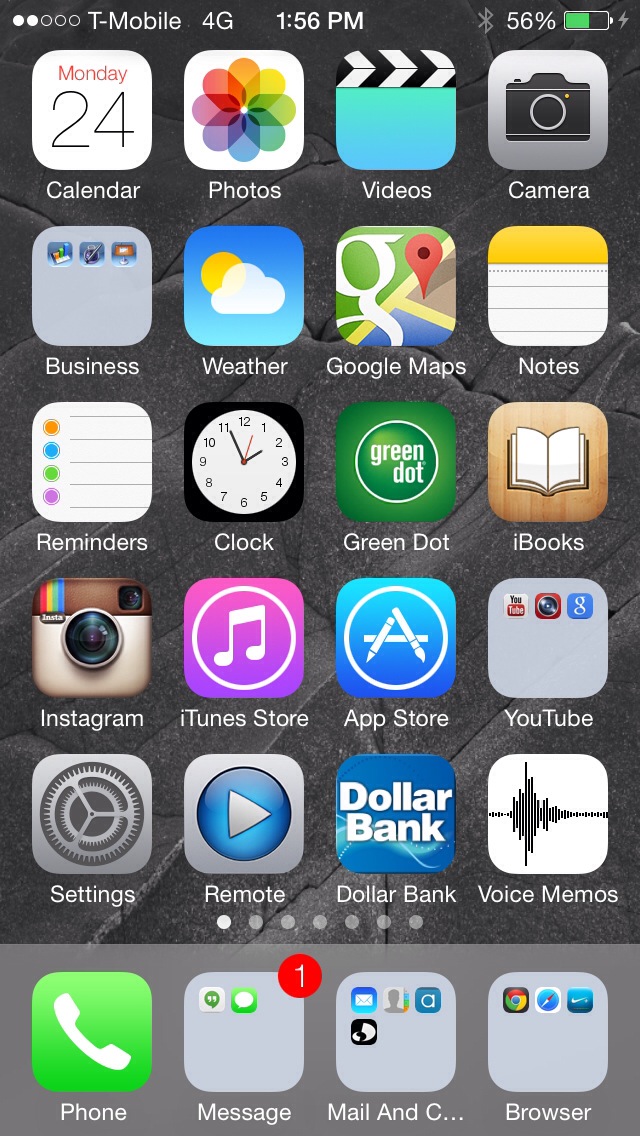A detailed photograph showcases a screenshot of an iPhone displaying the home screen. In the top-left corner, the T-Mobile network logo is visible alongside the 4G signal indicator. The time reads 1:56 p.m., with the battery level at 56%. The home screen is set against a dark background and populated with numerous apps.

Clearly visible are the Calendar app displaying the date as Monday the 24th, as well as the Photo, Video, and Camera apps. There is a business-related folder containing three apps. Additional apps include Weather, Google Maps, Notes, Reminders, Clock, Green Dot, iBooks, Instagram, iTunes Store, App Store, and YouTube, which is also grouped within a folder containing three apps. Settings, Remote, Dollar Bank, and Voice Memos are present as well.

At the bottom of the screen, the Phone app is positioned next to the Messages app, which shows one unread alert. Following this is a folder for Mail and another folder for Browser, which houses three apps.